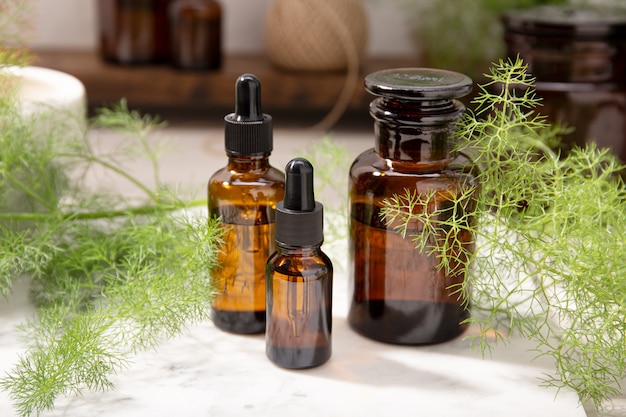This detailed photograph captures three small brown glass vials, prominently positioned on a crisp white surface. Two of the vials are fitted with eyedropper tops, while the third features a decanter-style stopper. Each vial contains a clear liquid, suggesting they hold essential oils or medicinal tinctures. Encircling the vials is a lush, vibrant green herb that appears freshly cut, adding a natural and wholesome element to the composition. In the softly blurred background, faintly outlined bottles on a shelf and a portion of a white bowl on the left contribute depth without detracting focus from the central subject. The image, with its emphasis on natural remedies and holistic wellness, could easily serve as an advertisement for essential oils or a promotional feature on a website dedicated to herbal products. The overall aesthetic is clean, organized, and vividly green, highlighting the purity and freshness of the contents within the vials.